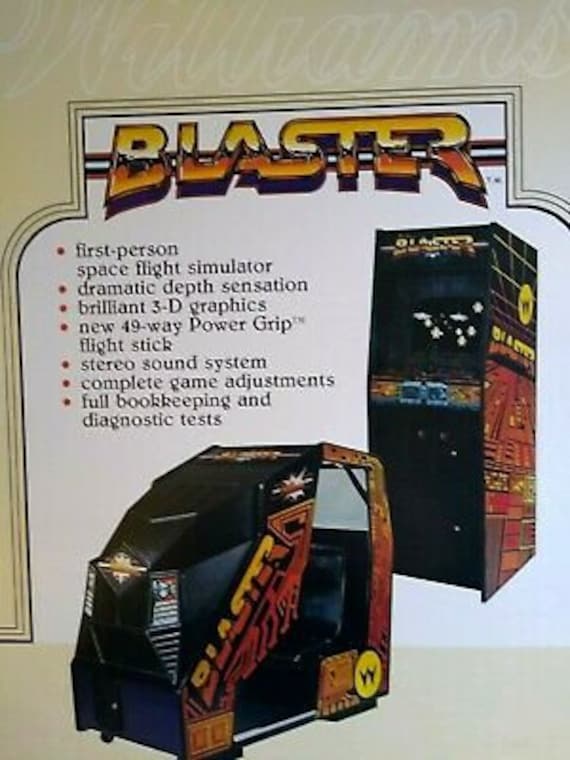This image depicts a vintage arcade game advertisement, evocative of the 1980s era. The flyer has a beige border and a tan upper section with a distinctive arch cut-out. In the top section, 'Williams' is faintly outlined in cursive. The central white portion features the title "Blaster" in large, futuristic yellow and orange letters.

Directly beneath the title are detailed bullet points in red with black text that highlight the game's features: 
- First Person Space Flight Simulator
- Dramatic Depth Sensation
- Brilliant 3D Graphics
- New 49-Way Power Grip Flight Stick
- Stereo Sound System
- Complete Game Adjustments
- Full Bookkeeping and Diagnostic Tests

The advertisement also showcases two different versions of the game – the standalone upright cabinet and the sit-down cockpit version. Both are adorned in matching colors of black, red, and yellow. The upright game has a traditional screen, joystick, and buttons setup, while the sit-down version offers an immersive playing experience where the player engages with the game from within an enclosed seat.